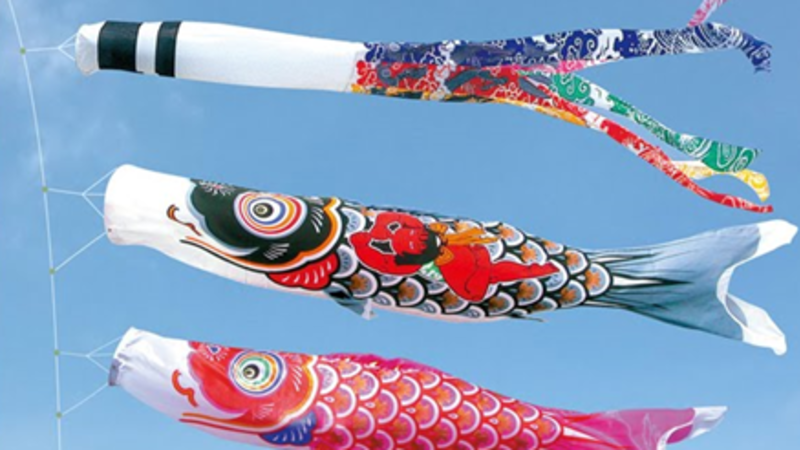The image captures a Japanese-style decoration of three fish-shaped kites, known as koinobori, fluttering horizontally against a clear blue sky with a few feathery white clouds on the left side. The kites are attached to a string on the left and facing right, their tails flowing in the wind. The top kite, designed to resemble a carp, has a white mouth and a body adorned with black and white stripes, followed by a multicolored tail featuring shades of blue, red, green, and yellow, spreading into four distinct strands. The middle kite is larger, with a white mouth and a large black head, transitioning into a body marked by gray and red scales, and ending in a gray and white tail. The bottom kite is predominantly pink, with a white mouth and tail, accented by hints of blue. All kites exhibit a tubular shape, enhancing their dynamic, wind-blown appearance in the bright and lively scene.